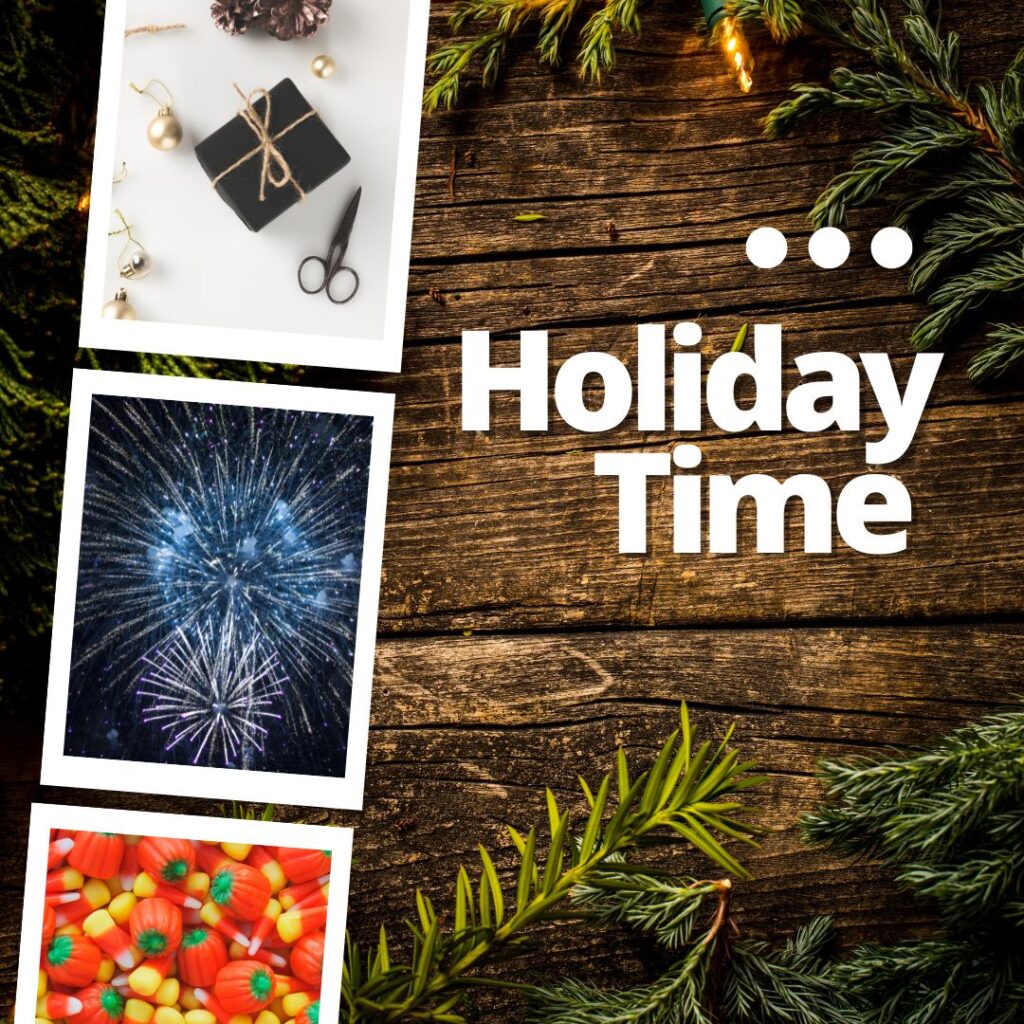The image features a rustic holiday theme set against a horizontally slatted wooden background with a rough, dark wood texture and pronounced grain, reminiscent of decking. Standing out in bold, white capital letters in the center, the text "HOLIDAY TIME" adorns the scene, accentuated by three white dots positioned above the D, A, and Y in "HOLIDAY." Surrounding the text and adorning the wooden backdrop are scattered pine needles and branches, creating a festive atmosphere akin to pine trees with a sprinkling of Christmas lights visible at the top.

To the left of the main phrase, three images are framed in white. The top image, slightly cut off, depicts a small, black present tied with a rope near a pair of black scissors and is accompanied by black and gold holiday ornaments. The middle image captures a vibrant display of fireworks, one blue and one white, set against a night sky. The bottom image showcases an assortment of Halloween-themed candies, including candy corn and candy pumpkins with green stems. Bright and clear, the overall image provides a well-lit and festive holiday setting.